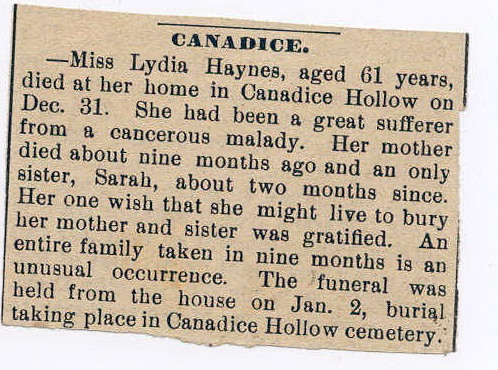This is an image of an obituary from a newspaper, showing a beige and black clipping. The obituary details the life and passing of Ms. Lydia Haynes, aged 61, who died at her home in Candace's Hollow on December 31st. Ms. Haynes was a great sufferer from a cancerous malady. Her mother passed away about nine months ago, and her only sister, Sarah, died about two months before her. Ms. Haynes' one wish to outlive her mother and sister so she could bury them was fulfilled. The entire family being taken within nine months is noted as an unusual occurrence. The funeral was held at her home on January 2nd, with the burial taking place in Candace's Hollow Cemetery. The layout of the text follows a standard newspaper format, positioned at an angle in the image and viewed from above.